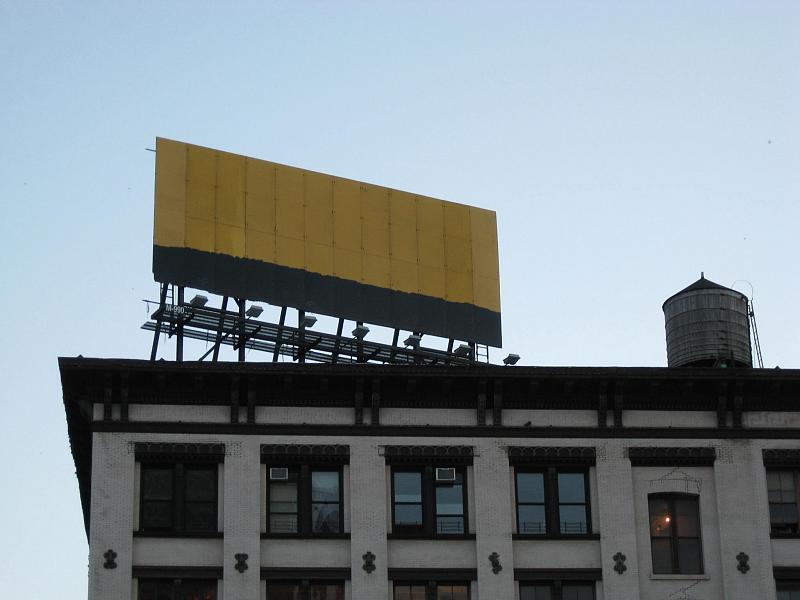The image captures a serene outdoor scene with a clear, light blue sky overhead, suggesting pleasant weather. Dominating the landscape is a prominent white building, its façade dotted with numerous windows. Notably, two of these windows are equipped with air conditioning units, which are black in color and mounted at the top. Perched on the top left corner of the building is a rectangular billboard, featuring a striking yellow color on its upper portion, adding a splash of vibrancy to the composed urban setting. The overall atmosphere is one of calm and clarity, with distinct structural details adding depth to the image.